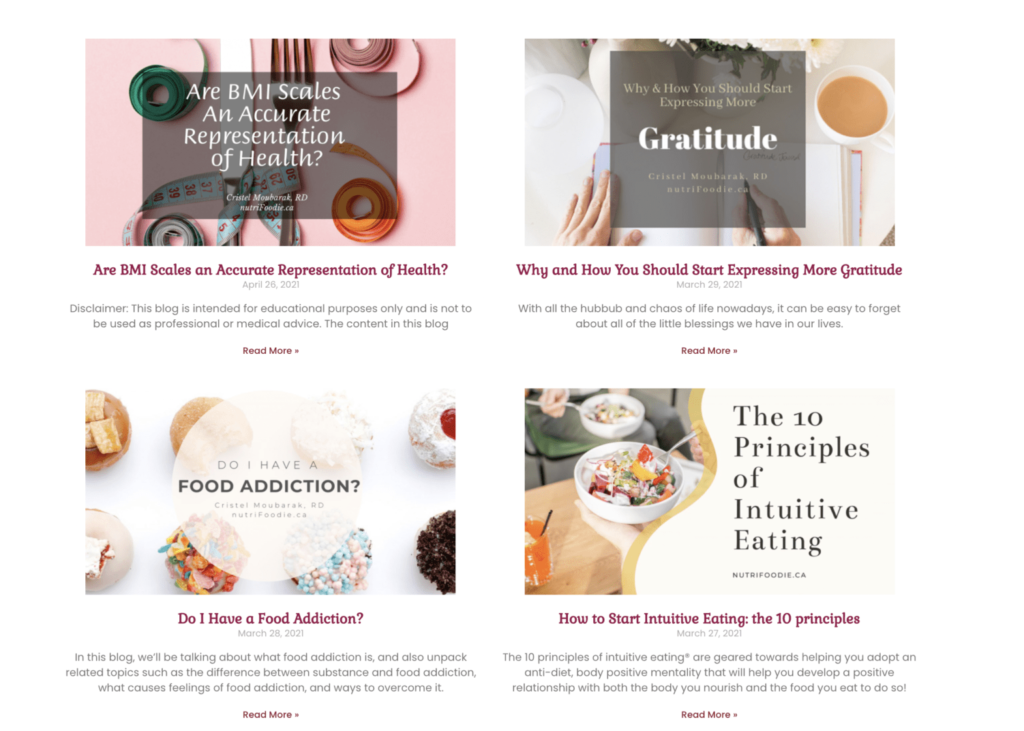This website features a well-organized layout with four distinct panels, each offering valuable content on health and wellness.

- **Top Left Panel:** Showcases a pink background adorned with measuring tapes, centered with a fork and knife, accompanied by a gray square. Inside the square, white text reads: "RBMI Scales and Accurate Representation of Health." Beneath this, in burgundy text, it repeats: "RBMI Scales and Accurate Representation of Health."
  
- **Top Right Panel:** Displays a cup of coffee and a person writing in a journal set against a darker gray background. The green text here says: "Why and How You Should Start Expressing More Gratitude." The word "Gratitude" appears in white text. Below, in burgundy print, it repeats: "Why and How You Should Start Expressing More Gratitude."
  
- **Bottom Left Panel:** Features various foods on plates, including donuts. The text here asks: "Do I Have a Food Addiction?" This is followed by the same question in burgundy text underneath: "Do I Have a Food Addiction?"
  
- **Bottom Right Panel:** Illustrates a graph on the left side, accompanied by images of two bowls and people sitting, with a gold line running through it. The text reads: "The 10 Principles of Intuitive Eating." Below, in burgundy text, it states: "How to Start Intuitive Eating: The 10 Principles," where "10" is represented as a numeral (1, 0).

Each panel effectively communicates its theme, providing a seamless and informative user experience on topics related to health, gratitude, food addiction, and intuitive eating.